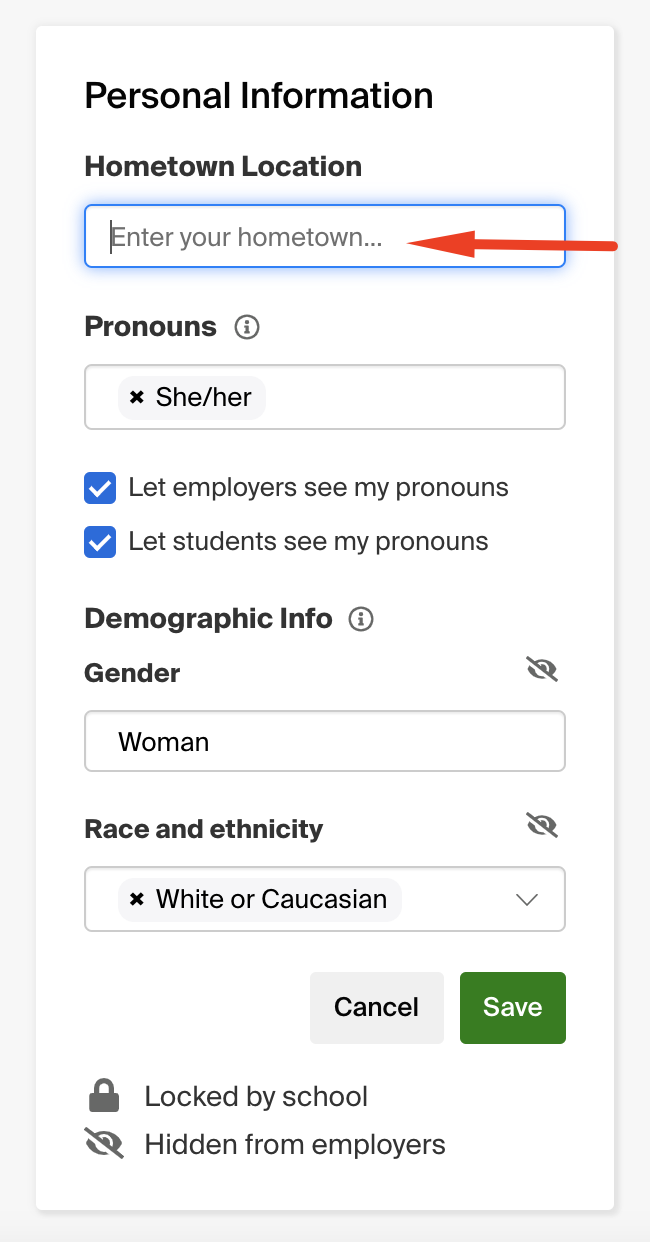The image is a screenshot designed to resemble a user interface on a smartphone. The background is completely white, contributing to a clean and simple layout. At the top, there is a header labeled "Personal Information." Below this header, there is a section titled "Hometown Location," with a text field where the cursor is positioned, ready for the user to enter their hometown. A striking red arrow points towards this search bar, drawing attention to it.

Further down, there is an option to select pronouns, with "She/Her" chosen from the available options. Directly underneath, there are two checkboxes labeled "Let employees see my pronouns" and "Let students see my pronouns," offering visibility options for the pronouns.

The next section is labeled "Demographic Information," where the user has entered their gender as "Woman." Below this, under "Race and Ethnicity," the user has selected "White or Caucasian." At the bottom of the screen, there are two buttons: a gray "Cancel" button on the left and a green "Save" button on the right, allowing the user to either discard or save their changes. Additionally, there is a small lock icon indicating that certain information is "Locked by School," and a note below stating that some information is "Hidden from Employers," signifying privacy settings in place.

Overall, the screenshot depicts a detailed and organized interface for updating personal, pronoun, and demographic information, with clear instructions and privacy options.